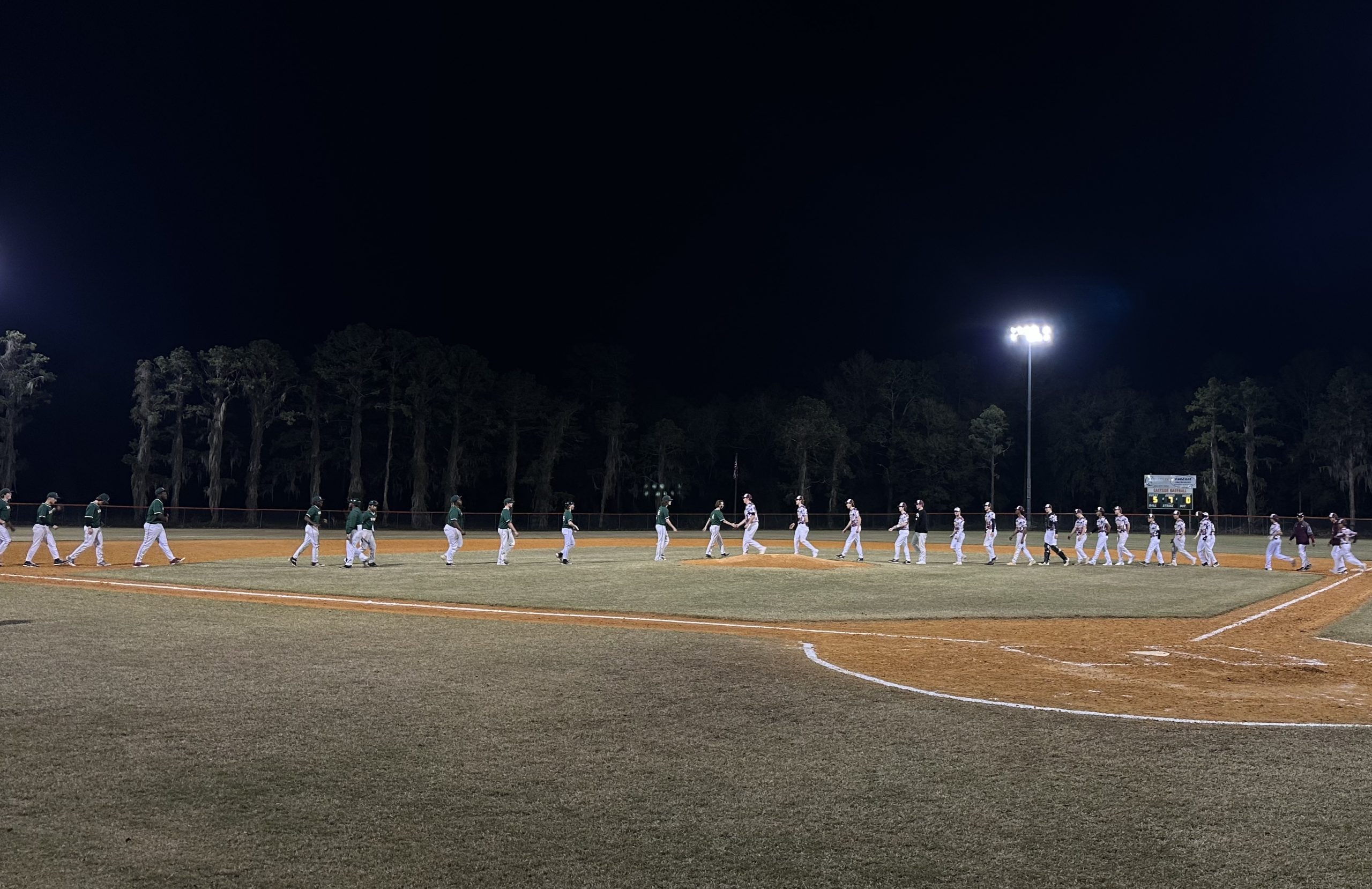As evening descends on a large baseball field framed by numerous trees in the background, two teams face each other, forming a line across the field from left to right. The sky is dark, illuminated by a single, large overhead light casting a soft glow over the scene. The players, identifiable by their jerseys, with one team in gray and the other in black or green, meet in the middle to shake hands, showcasing good sportsmanship at the end of the game. To the right of the field, a scoreboard stands sentinel, silently marking the conclusion of the match. The diamond, lined with white spray paint and interspersed with patches of grass, bears the marks of the game just played.